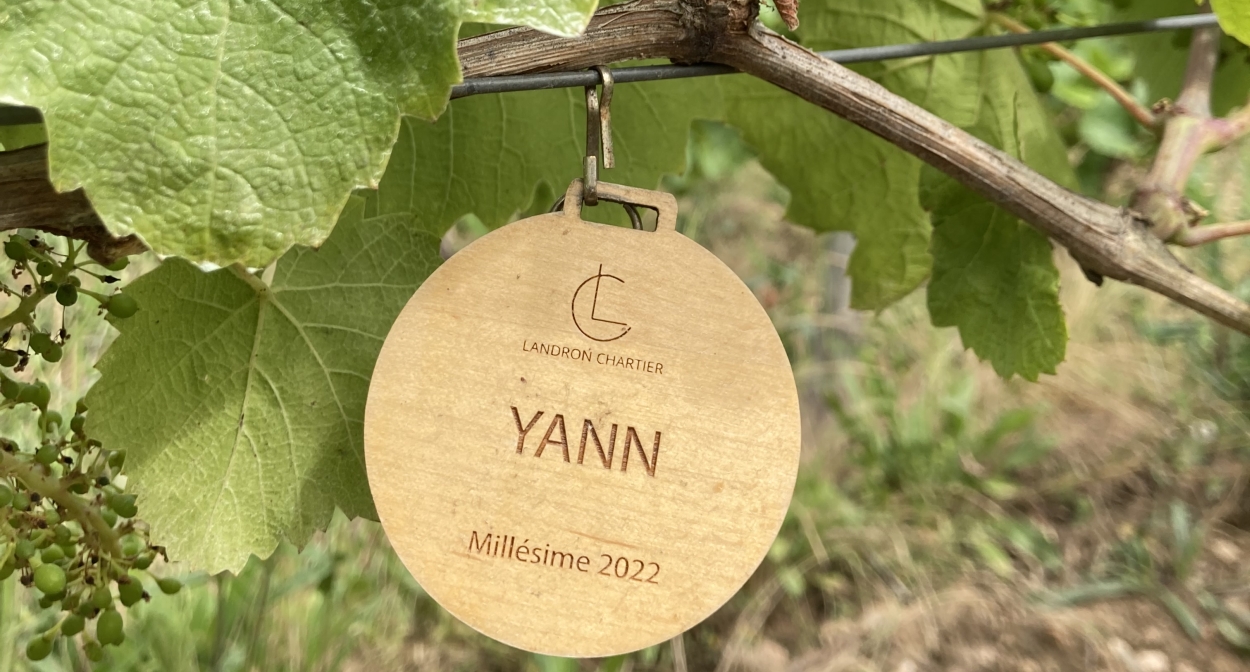This horizontally oriented outdoor photograph captures a picturesque grapevine setting. Spanning the top of the frame, a brownish vine is intertwined with a supporting wire fence. This vine is adorned with broad, bright green grape leaves, some of which hang down gracefully. Among the foliage on the left, small, immature green grapes can be seen, hinting at the promise of a future harvest.

Central to the image is a round, flat wooden placard suspended from the wire fence. The plaque features an intricately inscribed logo at the top, consisting of a thin 'C' and 'L' superimposed. Beneath this logo, the name “Landron Chartier” is elegantly carved. Dominating the center of the plaque is the name "YANN" boldly inscribed in large, thick capital letters. Below this, the text reads "Millésime 2022," indicating the vintage year of the grapes, and suggesting a connection to French winemaking traditions. The detailed craftsmanship of the carved letters adds a touch of rustic charm to this serene vineyard scene.